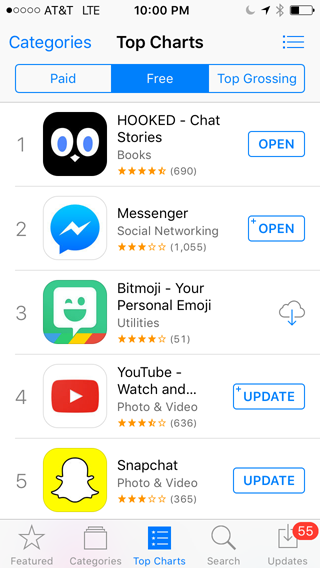This image is a screenshot of a cell phone display, showcasing a specific section of an app store.

At the top, there is a status bar containing five horizontal dots, with the first dot filled in black. To the right of these dots, it displays "AT&T LTE." The time is centered at "10:00 PM" in bold black text. On the far right of the status bar, icons include a grayed-out quarter moon, an upward arrow, a grayed-out Bluetooth symbol, and a battery icon showing about one-third remaining charge.

The top-left corner features the word "Categories" in sky blue. Centered below the status bar is the text "Top Charts" in black. On the far right, there is a menu icon consisting of three horizontal lines stacked vertically.

Directly beneath is a navigation bar divided into three sections. The left segment reads "Paid" in blue letters on a white background, the middle section shows a blue button labeled "Free" in white letters, and the right segment states "Top Grossing" in blue letters on a white background.

Below this navigation bar are several rows of app listings. The first app is labeled with a "1" and is named "Hooked - Chat Stories in Books," rated four and a half stars out of five. A blue horizontal button to the right says "Open." 

The second app is "Messenger - Social Networking," featuring the Facebook Messenger icon, rated three stars in yellow. A blue button on the right reads "Open."

The third app is "Bitmoji - Your Personal Emoji," rated four stars. Its icon displays a green and multicolored design, indicating it is in the cloud and needs downloading.

The fourth app is "YouTube," represented by the YouTube play button icon, with a three and a half star rating. The button on the right states "Update."

The fifth app is "Snapchat," identifiable by its ghost icon on a yellow background, rated three stars, with a right-side button labeled "Update."

At the bottom of the screen, a navigation bar features icons for "Featured" (a star), "Categories" (file folders), "Top Charts" (a list in blue), "Search" (a magnifying glass), and "Updates" (a square with a down arrow). The "Updates" icon includes a red bubble with the number 55.